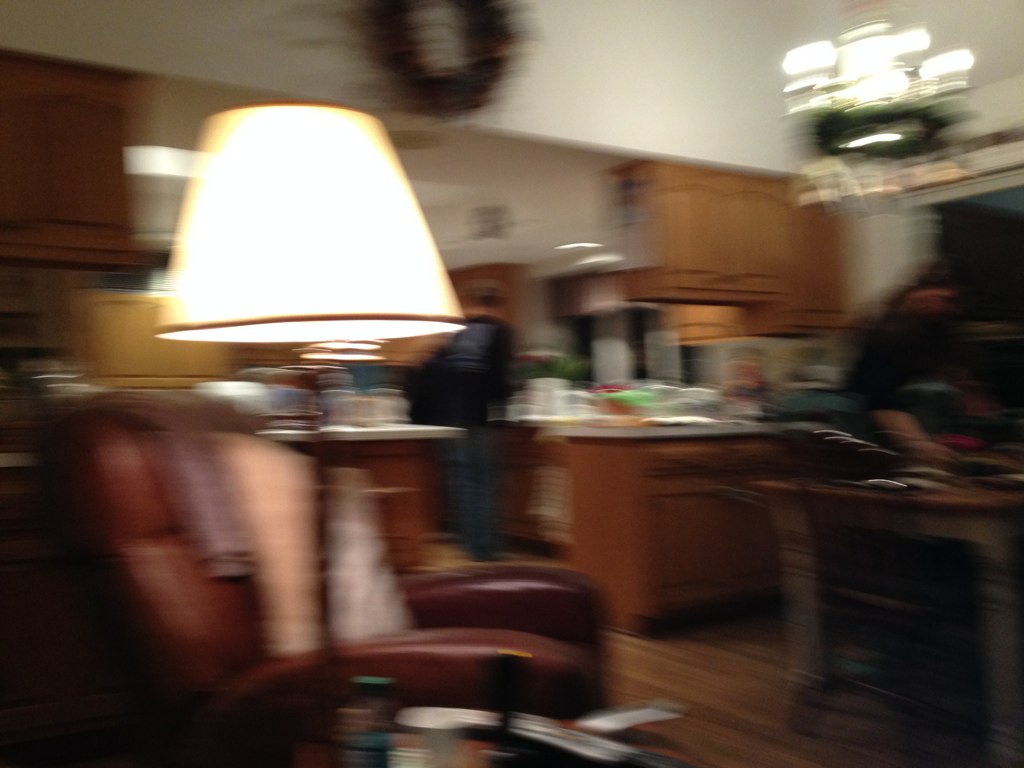In this blurry photograph, likely captured in motion, the viewer gets a glimpse into a cozy living room and kitchen area characterized by wooden floors. The image reveals a softly lit lamp and a comfortable chair anchoring the living room space. In the background, two individuals appear to be preparing a table, suggesting an element of domestic activity or meal preparation. The overall ambiance hints at a warm, lived-in home despite the indistinct and unfocused quality of the image.